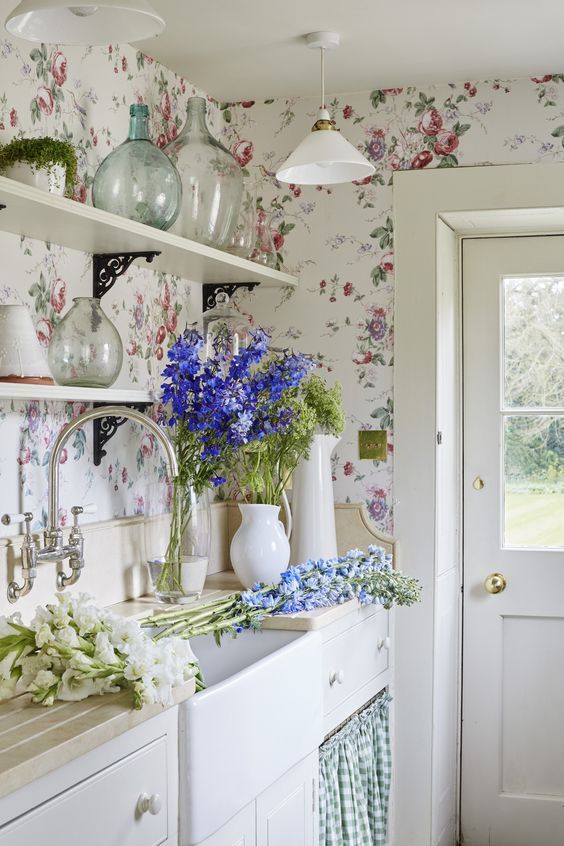The kitchen, adorned with white wallpaper featuring a vibrant pattern of red and purple flowers with green leaves, exudes a feminine touch emphasized by floral elements scattered throughout the interior. On the right side of the image, part of a white wooden door is visible, providing a glimpse of an inviting outdoor scene with lush green grass and several trees. Above, two pendant lights hang from the ceiling, each with a dome-shaped, upside-down cone design that holds light bulbs. 

In the middle of the picture, on the wall to the left, are two shelves displaying decorative glass containers, adding a touch of elegance to the space. Below the shelves is a white porcelain sink with a J-shaped, stainless steel faucet, set against a backdrop of cream-colored tiles. The countertop, which is wooden, supports a pot filled with blue and purple flowers, further enhancing the room's floral theme. Finally, the white cabinets below the counter and the overall white and cream color scheme tie the kitchen together in a cohesive and charming design.